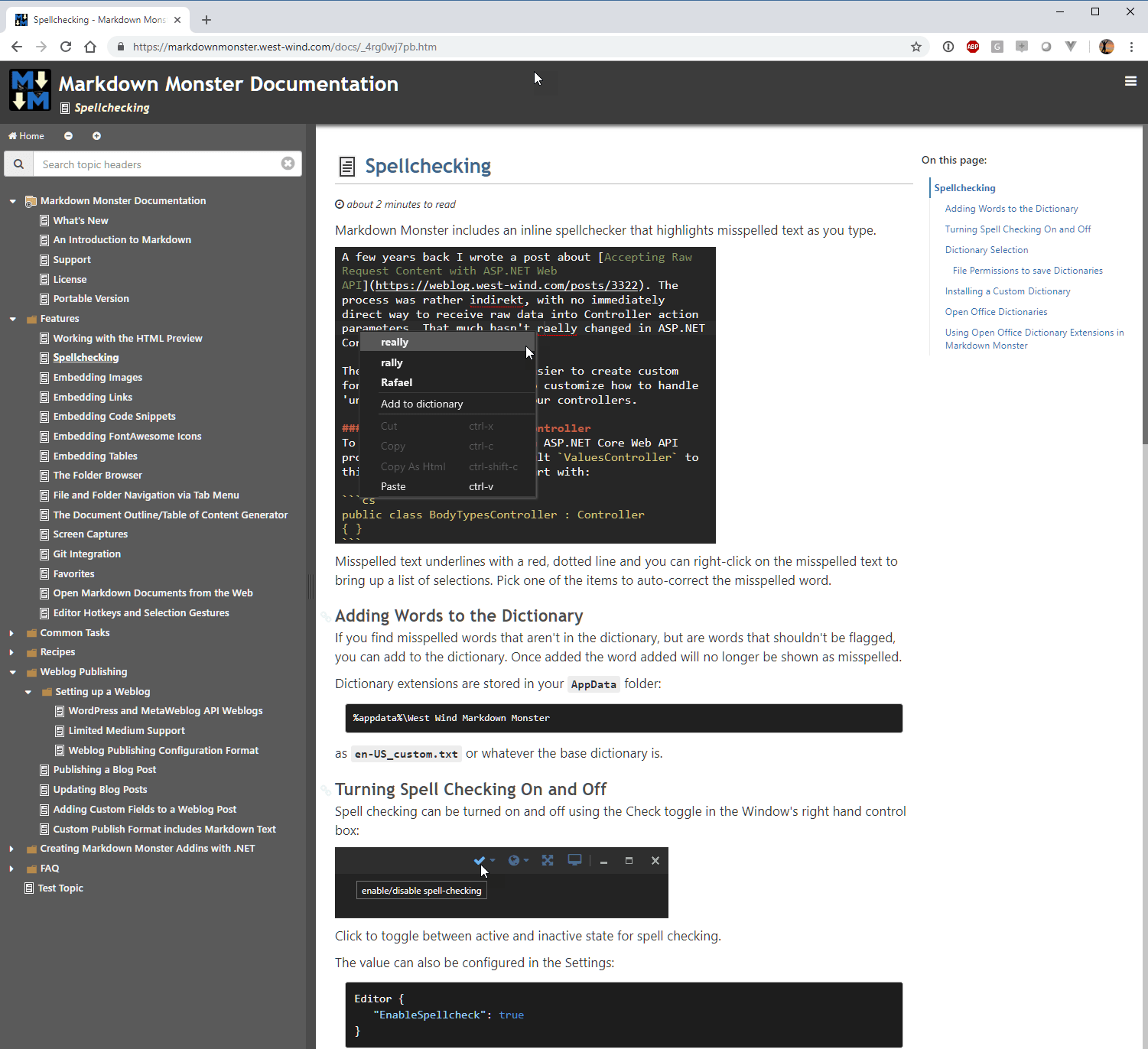This is a detailed screenshot of the Markdown Monster documentation webpage. The interface is displayed within a browser tab. The logo, displayed in the top left corner, is set against a black background. To its right, there are several navigational options and a search bar at the top for convenience. The left side of the page features a navigational panel with various subsections of the documentation.

The main content area is currently open to the 'Spellchecking' section, prominently displayed with the section title "Spellchecking" in blue in the top left of this area. Below this, the documentation states, "Markdown Monster includes an online spellchecker that highlights misspelled text as you type." There is an illustrative thumbnail depicting spellchecking in action, using the Slack web app as an example.

Further down the page, the documentation explains additional functionalities with sections titled 'Adding Words to the Dictionary' and 'Turning Spellcheck On and Off,' each accompanied by descriptive text and thumbnails.

To the extreme right of the page, there is a small section titled "On This Page" that provides quick links to various items described on the page, allowing for easy navigation within the documentation.